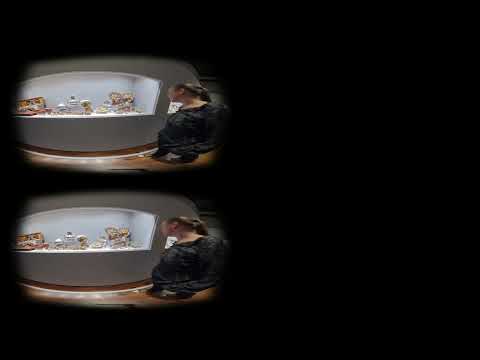The image is a horizontal rectangle predominantly shrouded in black. On the right side, the image fades into complete darkness, creating a stark contrast with the left side. The left half features two nearly identical, oval-shaped images stacked vertically with about two inches of space between them. These images are reminiscent of scenes viewed through an old-school TV monitor, with blurry edges enhancing this effect. 

Within each stacked image, the viewer's perspective is unusual, capturing a dimly lit interior space where individuals are walking or standing. In the foreground, a person stands with their back facing us, while another figure is walking toward the camera. Visible in the background are additional figures, partially obscured. The scene appears to take place in a room with a brown wooden floor, and through the windows within the images, some exterior buildings are visible.

The left side of the images also shows a rectangular cutout in a wall, illuminated to display several objects. This area is set into the wall, with bright lighting sharply contrasting the dim surroundings. The overall effect makes it seem as if the image was bordered or obstructed by an object, possibly a part of a hand, contributing to the segmented and layered visual experience.